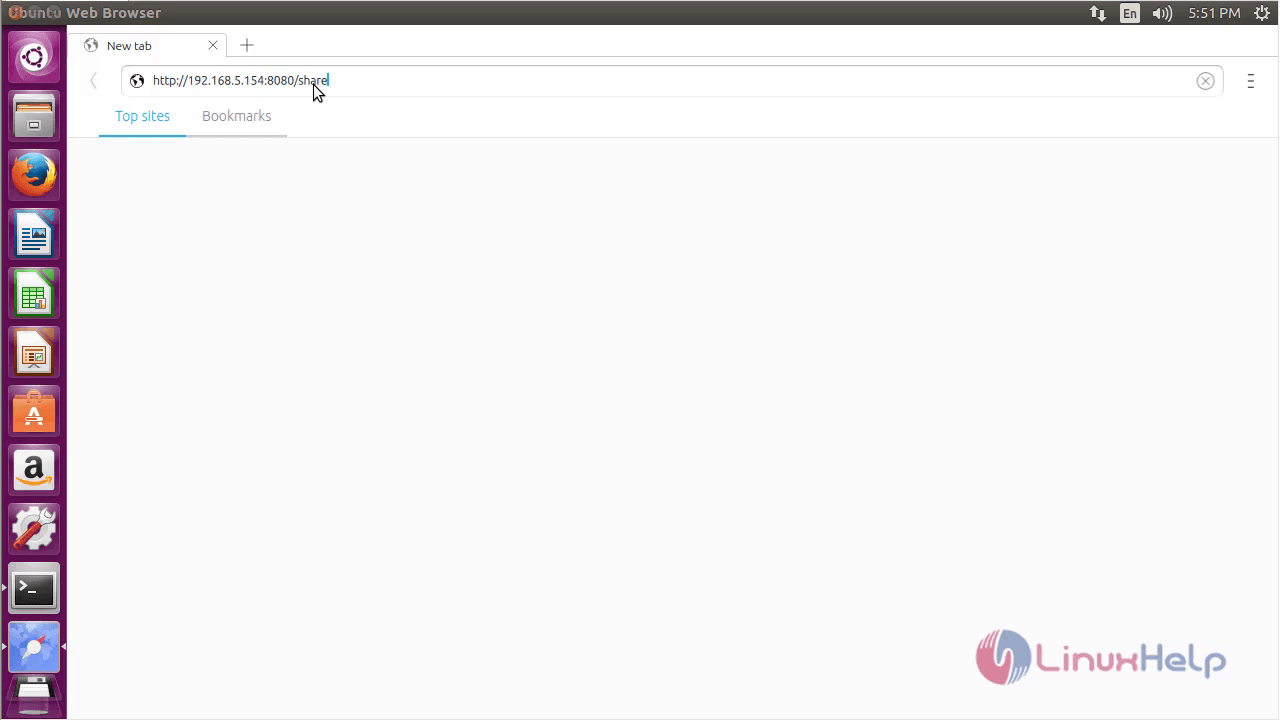The image shows a web page that appears to be related to Ubuntu, indicated by the branding at the top. The top banner prominently displays "B-U-N-T-U" in dark gray within a dark gray bezel, alongside the words "web browser" in white. To the right side, there are upward and downward white arrows, a white square with the letters "EN" in black, a speaker icon emitting white waves, and the current time displayed as "5:51 PM". Additionally, there's a white gear symbol for settings.

On the left side of the banner, there is a purple square with violet bands and a dark purple gear with some white accents beside it. Below are several application icons: 
- A dark gray folder icon with tan and brown inner folders.
- The Firefox logo featuring an orange and yellow fox encircling a blue globe.
- A white web page icon with lines of black text and dark blue accents.
- An Excel-like green icon with white details.
- A PowerPoint-like icon that is tan with red and blue bands, set against a white background.
- An orange briefcase icon with an "A" and orange bands.
- The Amazon logo, a white square with a lowercase black "a" and an orange swoosh arrow.
- A gray gear icon intersected by a wrench that fades to red.
- A dark gray computer terminal displaying a black interior, a white cursor arrow, and a white border.
- A dark gray square containing light and dark blue patterns, a white circle, and an orange circle.
- A purple drawer icon featuring a black floppy disk with a white label and silver top within a white area.

The active browser tab shows a globe icon next to the title "New Tab" with a plus sign and a left-pointing arrow. The URL displayed is "https://192.168.5.154:8080/SHARE" with a blue pointer icon next to it. The web page has a white background with cyan blue highlighted text and an underline for "Top Sites", though no sites are listed. The "Bookmarks" label is gray with a gray underline.

In the lower-left corner, there is a circular icon with a red and blue hand, labeled "Linux HELP" with "Linux" in red and "HELP" in blue, with capitalized "H" and "L".